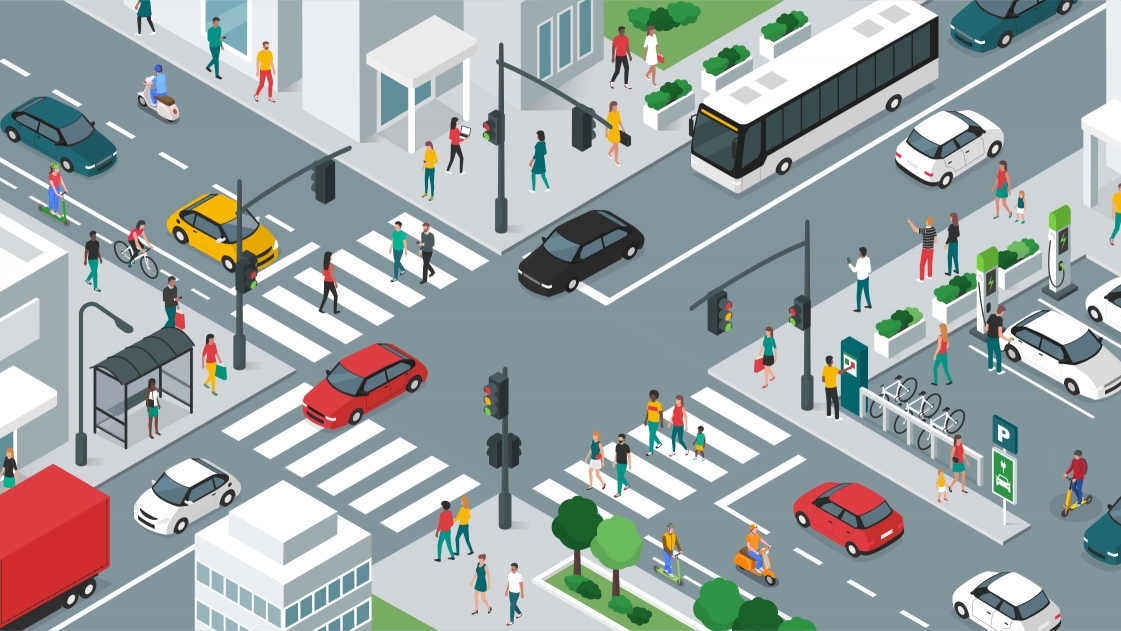This vibrant, hand-drawn, color cartoon illustration depicts a bustling city intersection viewed from a 45-degree angle, resembling a drone shot. The scene features two city streets crossing diagonally from the upper right to the lower left, and from the upper left to the lower right, forming an X. The streets are rendered in gray with detailed crosswalks.

At the intersection, traffic with a green light flows from the upper right corner to the bottom left, comprising a large red truck, a white car, a red car, and a black car, followed by a white bus with black-trimmed windows. On the opposite diagonal route, halted by a red light, vehicles await their turn. Streetlights adorn both corners of the crosswalks, enhancing the urban ambiance.

The sidewalks on either side of the street are animated with cartoon pedestrians. Some stand waiting to cross, while others are already making their way across the crosswalks. On the lower left corner, a bus stop shelter with a person inside awaits the approaching bus. The right corner features a paid parking lot with a row of bicycles and flower boxes with greenery, adding a touch of nature to the cityscape. Several buildings frame the scene, completing this lively urban tableau.